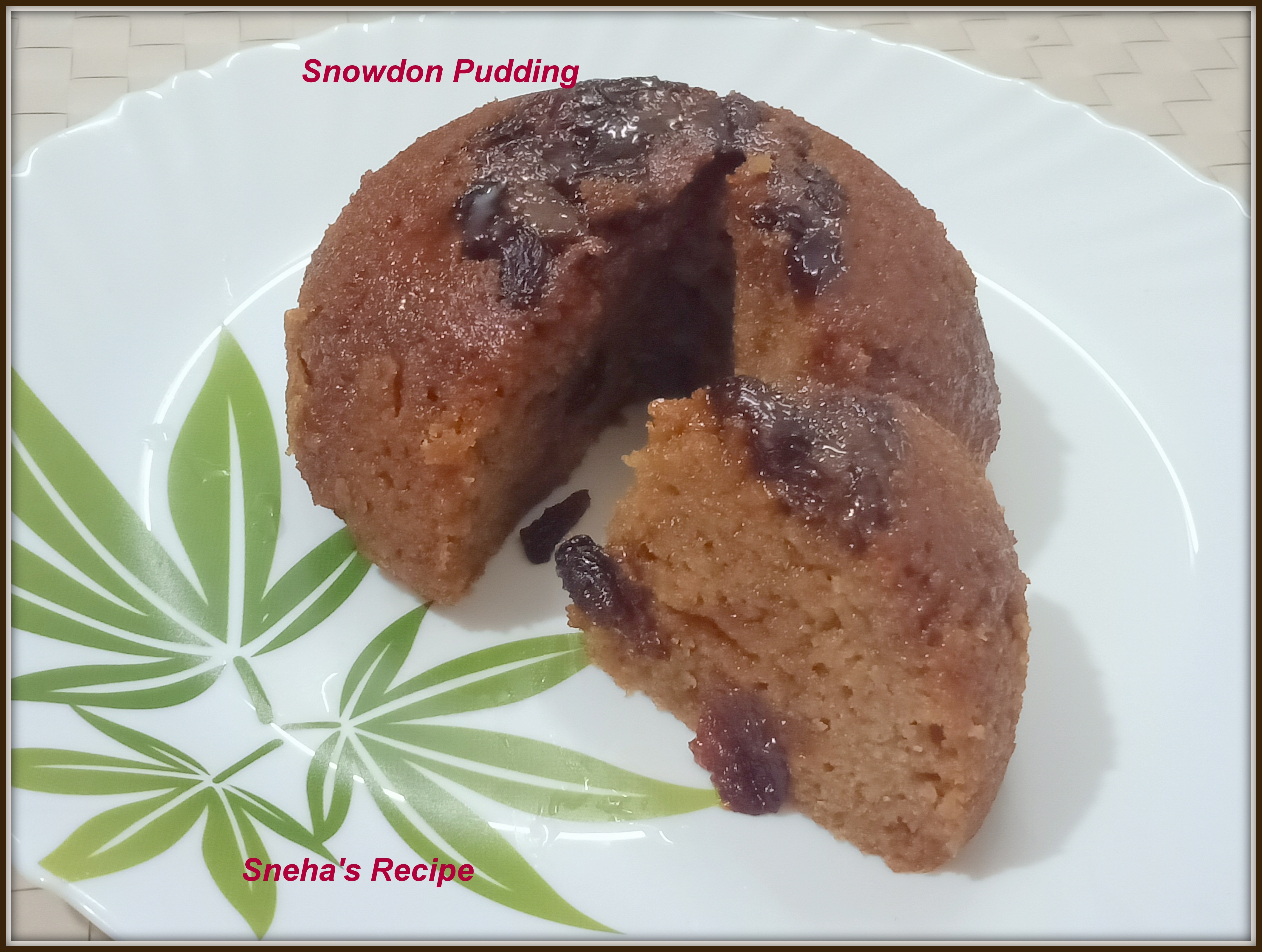The image depicts a circular Snow Don Pudding, moist and glazed, showcased on a glossy white plate adorned with green leaves that resemble cannabis in the bottom left corner. Red text reading "Sneha's Recipe" is distinctively positioned on the bottom left of the plate, while the top of the image features the text "Snow Don Pudding." The pudding, brown in color and embedded with raisins, has a slice neatly cut out, revealing a rich internal texture. Raisins are predominantly seen on the top of the pudding and have also fallen onto the plate. The plate covers most of the frame, resting on a light brown, textured surface. A zigzagging pattern can be observed in the background, formed by tiles. The source of light is from the left, casting a shadow of the pudding to the right, enhancing the visual depth of the scene.